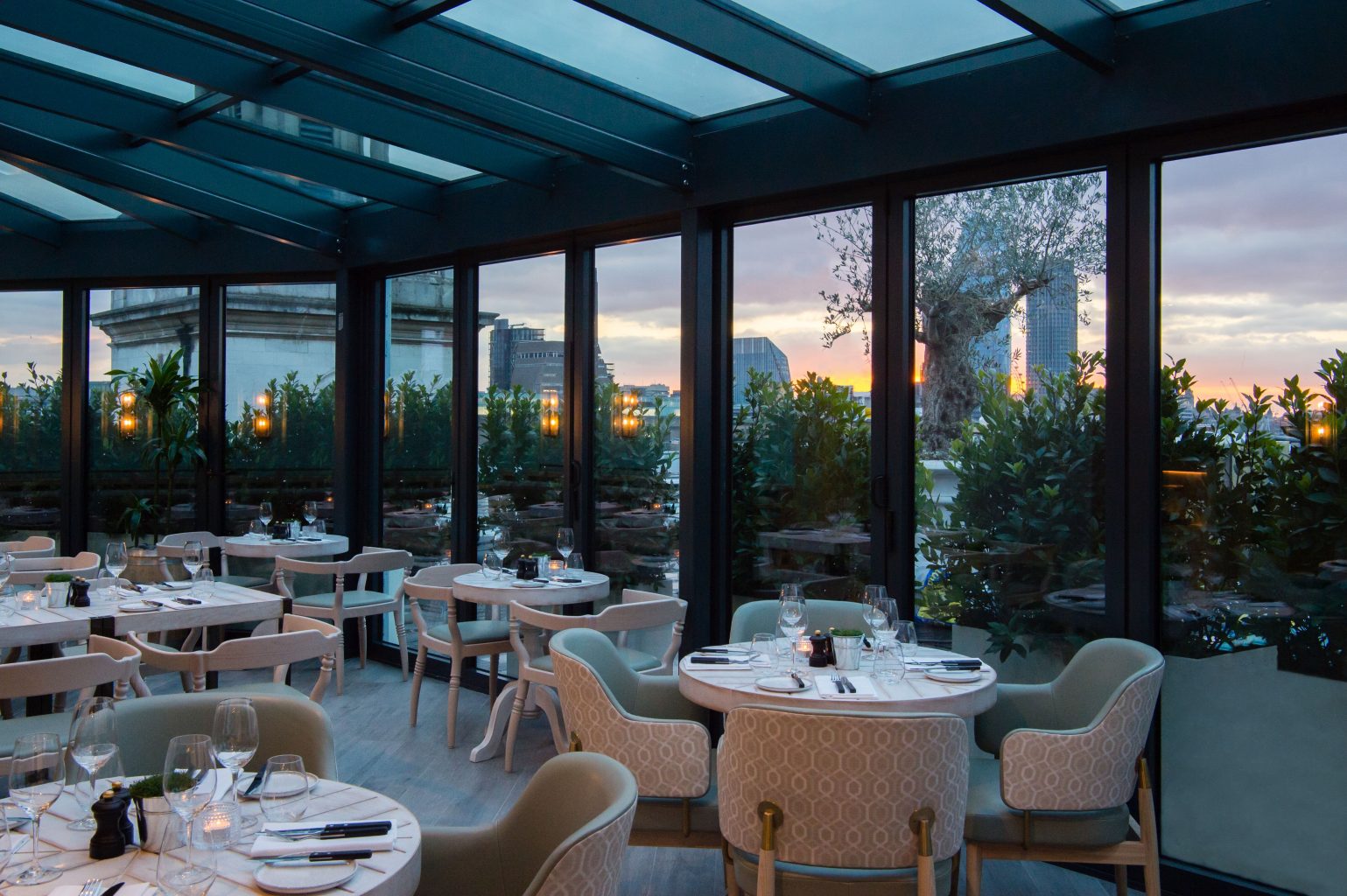This professional photograph captures the serene ambiance of an indoor dining area within a restaurant designed like a sunroom or veranda. The space is uniquely surrounded by floor-to-ceiling glass walls and a mostly glass roof, supported by metal beams, allowing abundant natural light to flood the interior. This structural design offers diners a panoramic view of a lush outdoor garden with trees, flowers, bushes, and distant, aesthetically pleasing buildings, including skyscrapers. 

The dining area features round tables, predominantly designed for two or four patrons. Each table is elegantly set with wine glasses, fine china, silverware, napkins, and candles, suggesting a high-end dining experience. The chairs, covered in a soft beige upholstery with decorative patterns, provide a cozy seating arrangement. Some descriptions mention chair interiors with a hint of teal, emphasizing the restaurant's attention to detail and design. 

The photograph is likely taken during sunset, as indicated by the warm orange and purple hues near the horizon transitioning into a deep blue sky above. The absence of diners and the meticulous table settings suggest that this image was captured during off hours, possibly for promotional purposes. The overall color palette includes black, white, grey, brown, beige, green, orange, purple, red, and blue, adding to the visual richness of the scene.